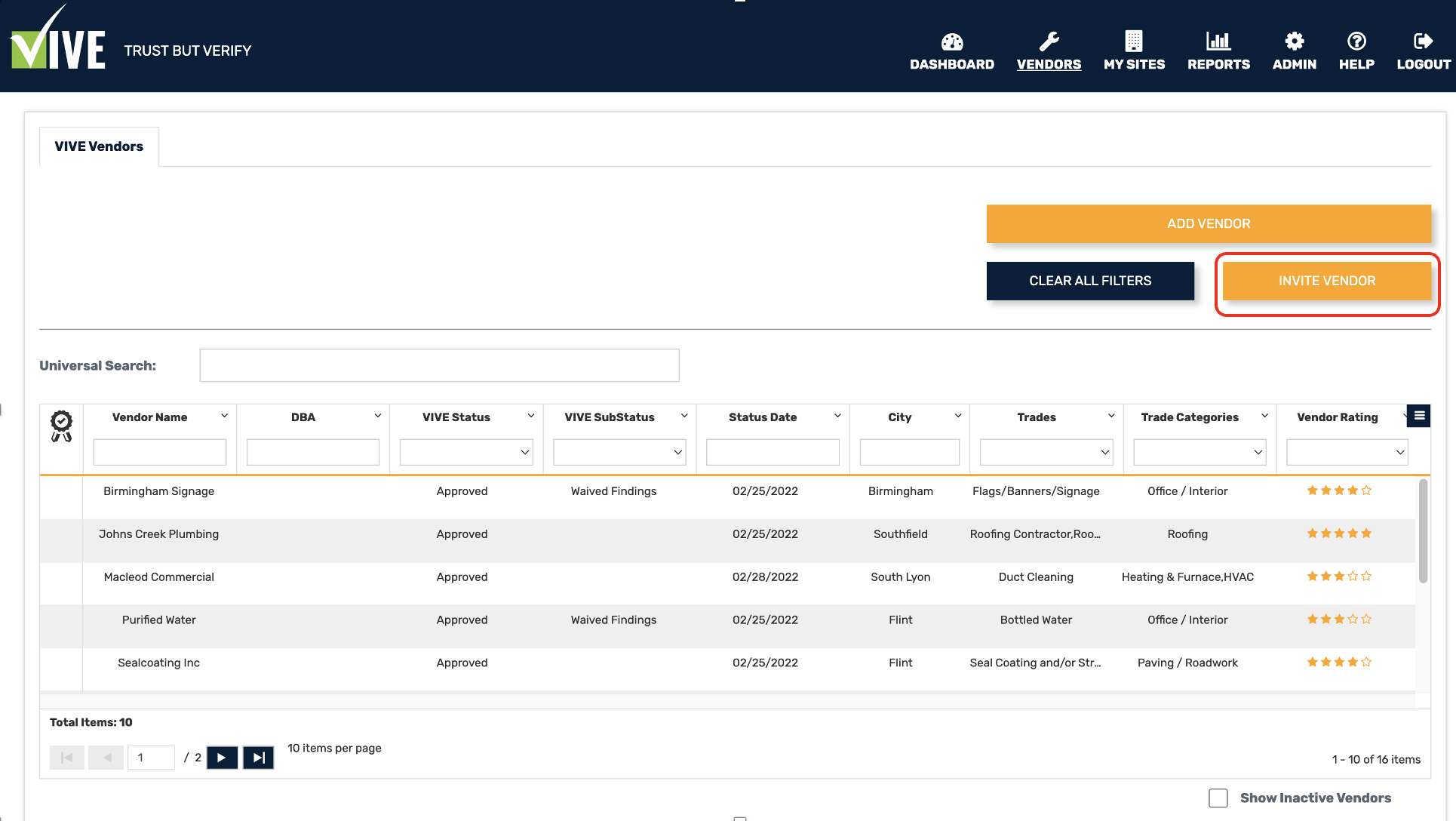This image is a detailed screenshot of the VIVE dashboard interface, accompanied with the slogan, "Trust but Verify," prominently displayed at the top. The word "VIVE" is enclosed in a green box, with the 'V' stylized as a white checkmark, followed by the letters 'IVE' in white uppercase text. 

In the top-right corner of the banner, several navigation options are available: Dashboard, Vendors, My Sites, Reports, Admin, Help, and Logout.

Below the main banner, there are buttons labeled "VIVE Vendors," "Add Vendor," "Clear All Filters," and "Invite Vendor," with the "Invite Vendor" option currently selected.

The search and filter section includes categories such as Universal Search, Vendor Name, DBA (Doing Business As), VIVE Status, VIVE Substatus, Status Date, City, Trades, Trade Categories, and Vendor Rating. 

Beneath this, a list of approved businesses is displayed with specific details:

1. **Birmingham Signage**
   - Status: Approved
   - Substatus: WAVED Findings
   - Date: 2-25-2022
   - Location: Birmingham
   - Categories: Flags/Banners/Signage, Office/Interior
   - Rating: 4 out of 5 stars

2. **Johns Creek Plumbing**
   - Status: Approved
   - Date: 2-25-2022
   - Location: Southfield
   - Categories: Roofing Contractor, Roofing
   - Rating: 5 stars

3. **MacLeod Commercial**
   - Status: Approved
   - Date: 2-28-2022
   - Location: South Lyon
   - Categories: Duct Cleaning, Heating and Furnace/HVAC
   - Rating: 3 out of 5 stars

4. **Purified Water**
   - Status: Approved
   - Substatus: WAVED Findings
   - Date: 2-25-2022
   - Location: Flint
   - Categories: Bottled Water, Office/Interior
   - Rating: 3 stars

5. **Seal Coating, Inc.**
   - Status: Approved
   - Date: 2-25-2022
   - Location: Flint
   - Categories: Seal Coating and/or Paving/Roadwork (partially cut off)
   - Rating: 4 out of 5 stars

This screenshot provides a comprehensive view of the vendor management and status tracking system within the VIVE platform.